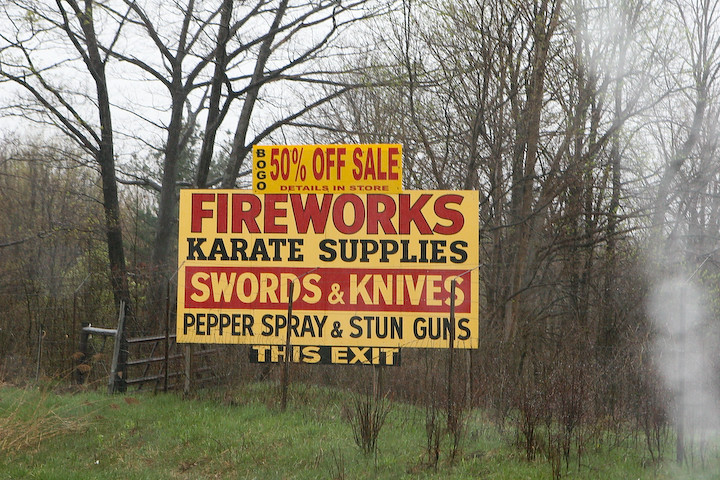In this image, we see a large yellow sign positioned at the edge of a leafless forest, implying that it might be winter. The sky is grey, creating a somewhat somber backdrop. The ground features patches of green grass and some bushes at the base of the sign. To the left, there is a brownish-grey fence and a larger tree among several other barren trees. 

The sign is held up by two poles and topped with a bright yellow section that advertises a "BOGO, 50% off sale, details in store." Below this, the main part of the sign lists various items: "Fireworks" in red letters, "Karate Supplies" in black, "Swords and Knives" displayed on a red background in white lettering, "Pepper Spray and Stun Guns" in black letters, and at the bottom with a black outline in white and yellow, it reads "This Exit," hinting that the advertised items can be purchased nearby.

The overall setting is slightly foggy to the right, further enhancing the isolated and mysterious atmosphere of the image.